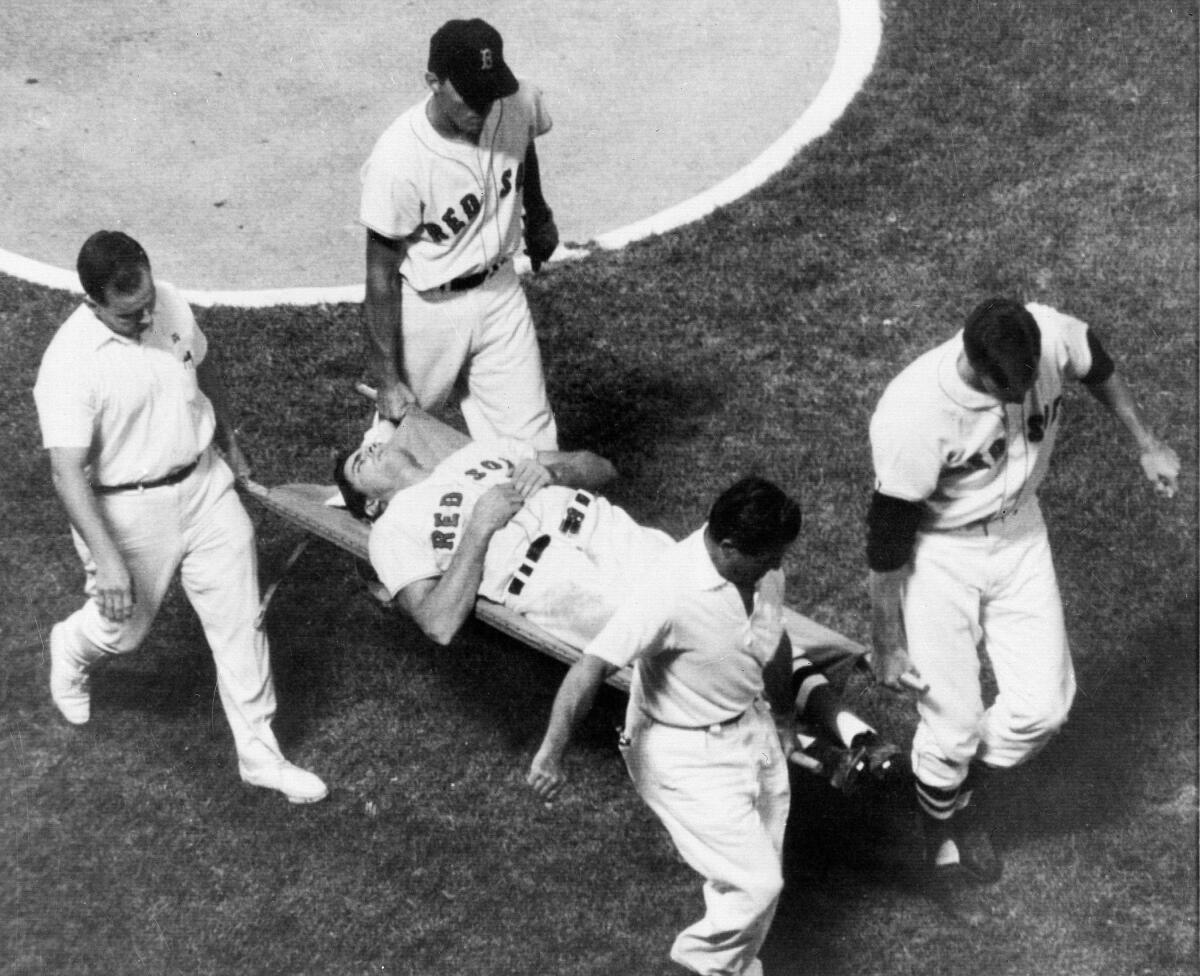This black-and-white photograph captures a poignant moment during a baseball game featuring the Boston Red Sox. The image displays five men: a Boston Red Sox player lying on a stretcher being carried off the field by two fellow Red Sox players and two medical personnel. The player on the stretcher is dressed in a light-colored uniform with "Red Sox" emblazoned across his chest, and his hands rest on his stomach with his face turned upwards and eyes closed. His belt appears to be unbuckled, indicating he was likely injured during the game.

The stretcher is composed of canvas material and supported by wooden poles. Each of the four men is grasping a corner of the poles: two Red Sox players on the right, identifiable by their team uniforms and the fact that they are holding their hats, and two medical staff members on the left, wearing white tops, trousers, and white sneakers. The setting is on a grassy field, with a circular, light-colored area bordered by a white trim visible in the background, suggesting an outdoor location, possibly near the baseball diamond or a parking lot.